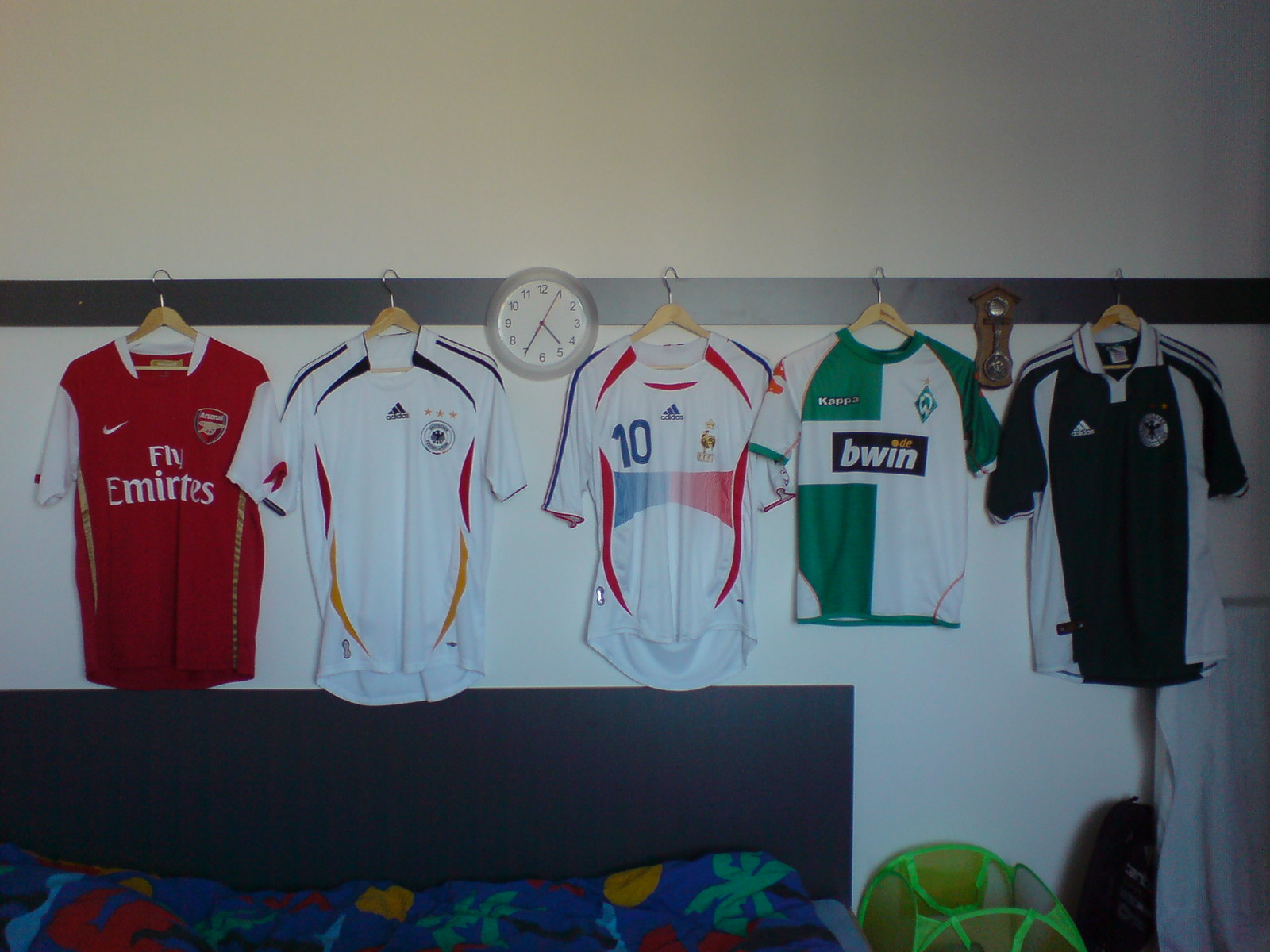The photograph depicts a section of a wall that is half beige at the top and half white at the bottom, divided by a dark strip which appears to be metal. Five soccer jerseys are meticulously hung on wooden hangers from this dark strip, each jersey displaying distinct colors and patterns. From left to right, the jerseys are: predominantly red and white emblazoned with “Fly Emirates,” a white jersey with black, red, and yellow stripes, a white jersey featuring number 10 with blue and red stripes, a green and white jersey with “Bwin,” and finally, a black and white jersey. In front of the jerseys, an analog clock with the time 5:35 is mounted on the wall, positioned between the second and third jerseys. Below the jerseys, at the bottom of the wall, there’s a blue blanket adorned with yellow, light green, and red designs, and to its right, a neon green fabric or small hamper. The detailed background includes a continuation of the white wall and a dark gray squared pattern near the bottom left-hand side, adding texture to the setting.